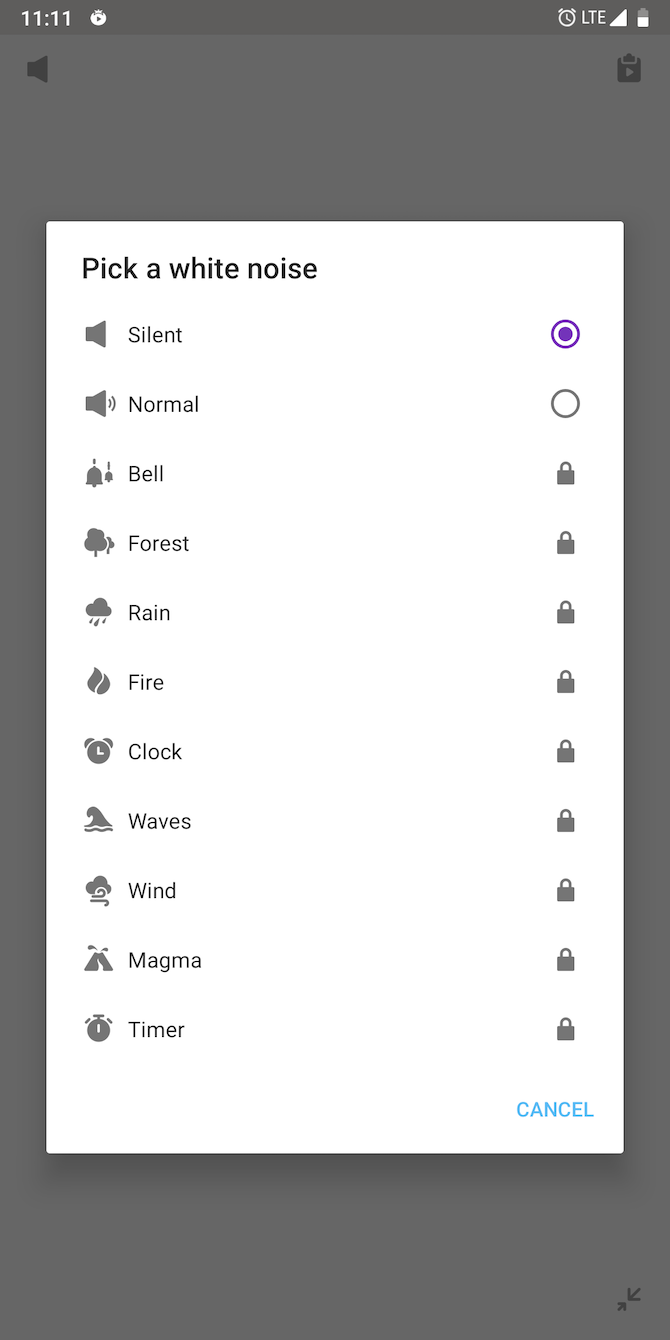This image depicts a smartphone screen with a detailed user interface related to selecting white noise sounds. The phone displays an LTE signal and a battery life at approximately 75%, with the current time shown as 11:11. In the upper portion of the screen, there is an icon indicating the phone is in silent mode. 

Central to the screen is a prominent pop-up box titled "Pick a White Noise," with "Silent" currently selected. The "Silent" option is represented by a small purple circle, both outlined and filled with purple. Beneath this, the text "Normal" appears with its corresponding icon, showing sound waves emanating from a circle; this icon is white and unselected.

Below the "Normal" option, there are multiple white noise selections, each accompanied by a lock icon indicating their inaccessibility. These options include "Bell," "Forest," "Rain," "Fire," "Clock," "Waves," "Wind," "Magma," and "Timer." Each locked icon is a black padlock. 

At the bottom of the pop-up box, a "Cancel" button is highlighted in a soothing teal blue shade. The background of the screen beneath this pop-up is a continuous gray.